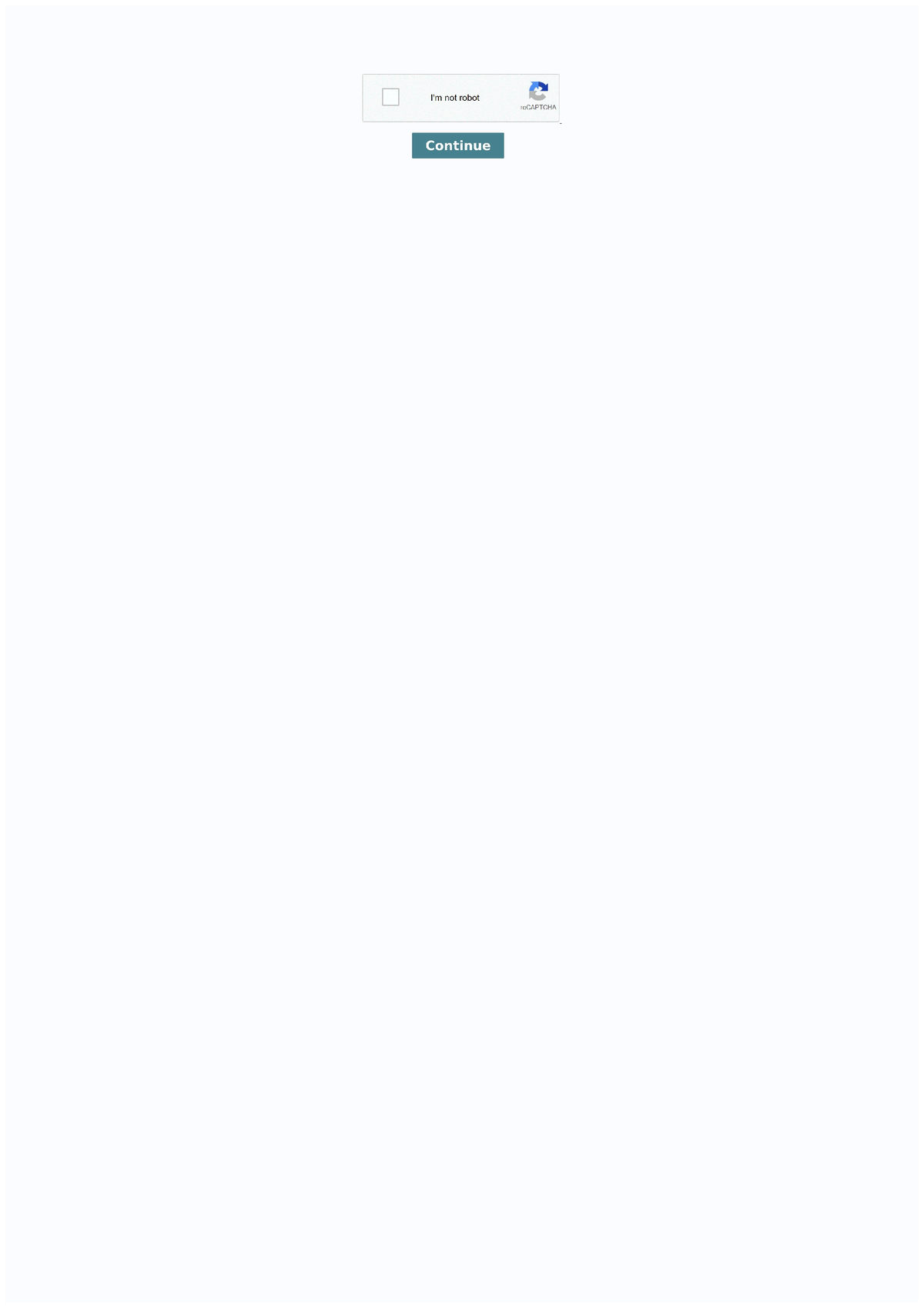The image showcases a CAPTCHA verification screen, commonly seen on login pages to distinguish human users from automated bots. The overall background is a very light gray, almost off-white. Centered at the top of the screen is a light gray rectangle bordered by a slightly darker gray, yet still light, border. 

To the left within this rectangle is a white square, similarly bordered by the same dark light gray. Inside this square, the text "I'm not a robot" is displayed in black Arial font, which gives a clean, sans-serif appearance. 

Adjacent to the text, on the right side, is the recognizable CAPTCHA symbol, featuring a gray curved arrow that transitions into a light blue and then a dark blue arrow. Beneath this symbol, the letters "e" (lowercase) and "CAPTCHA" (uppercase) are printed in black.

Below the CAPTCHA verification section is a dark teal rectangular button. Centered on the button, the word "Continue" is boldly written in white font, indicating the action to move forward once the user has selected the tick box proving they are human.

This section occupies a small top portion of the overall page, which is described as very long and rectangular. The CAPTCHA and associated elements take up less than one-tenth of the entire page.